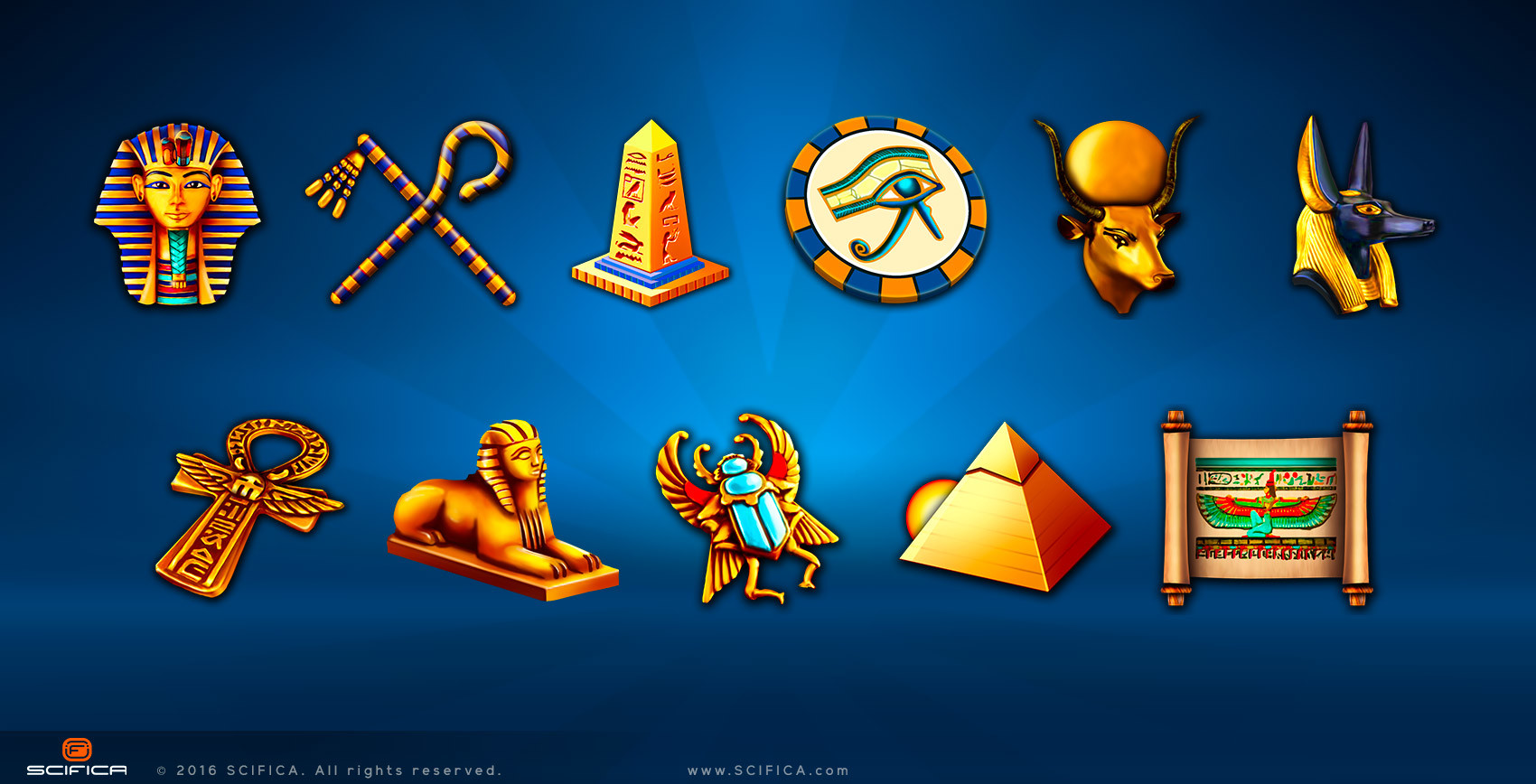The image features a blue background adorned with about a dozen ancient Egyptian-inspired icons arranged in two rows. In the top row, from left to right, there is a pharaoh's tomb head, a set of crossing canes, a pyramid-shaped monument, a coin with an eye, a cow's head with horns and a golden ball, and an Anubis figure. The bottom row includes icons of an ankh, a sphinx, a turquoise scarab beetle with gold legs and wings, a golden pyramid, and a scroll featuring an Aztec bird symbol. The lower left corner of the image displays the website www.scifica.com, the Scifica logo, and the text "© 2016 Scifica. All Rights Reserved."